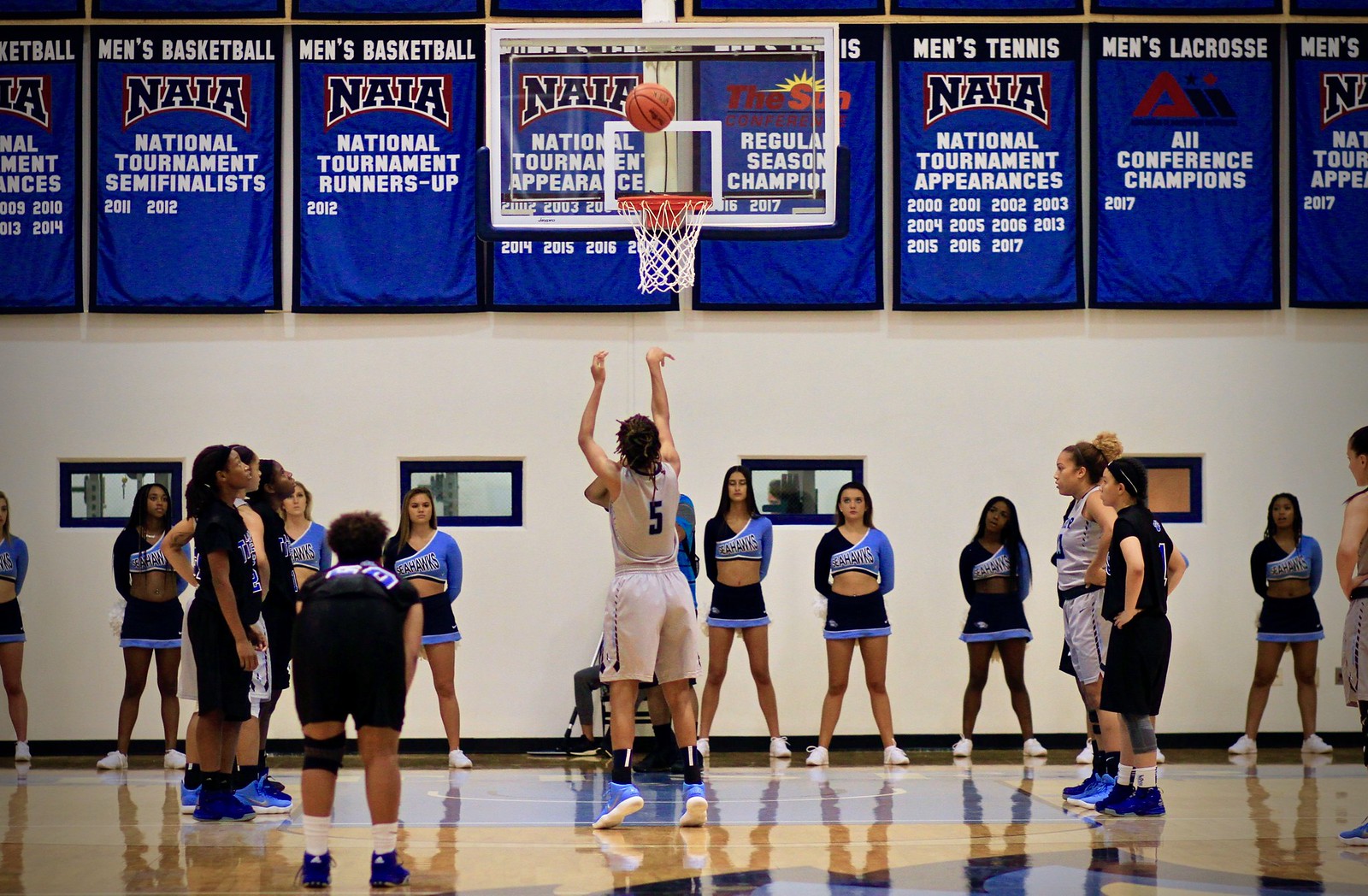This color photograph captures a tense moment in a women's basketball game, portraying the scene from center court facing the basketball goal. Central to the image is player number five, dressed in a beige jersey and white shorts with black socks and white high-top sneakers, poised at the free throw line. The basketball, suspended midair just above the basket, hints at the delicacy of the moment. Surrounding the shooter, players stand ready, characterized by their black jerseys, black shorts, and dark blue shoes.

Behind the translucent backboard, the white wall adorned with small windows and numerous championship banners adds a storied backdrop. These blue banners commemorate the accolades of men's basketball, tennis, lacrosse, and football teams, showcasing various achievements and tournament placements.

Additionally, the presence of cheerleaders, all dressed in matching dark blue and light blue uniforms with white sneakers, brings extra vibrancy to the scene. Positioned at parade rest against the back wall, they attentively observe the proceedings. The polished wooden court, accented with blue paint, completes the vivid and dynamic atmosphere of the indoor arena.